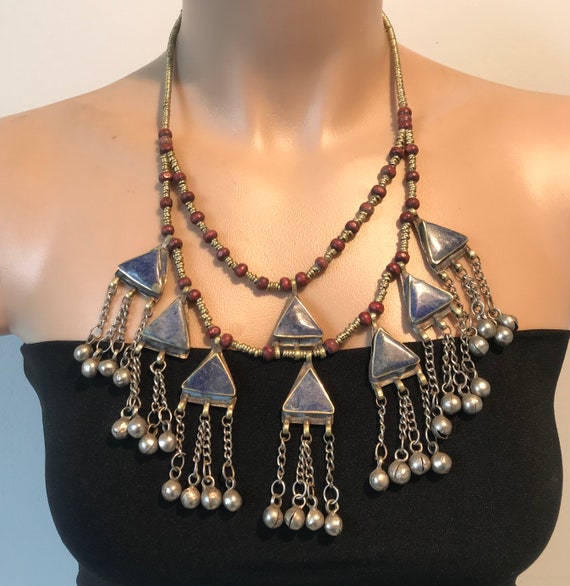The image depicts a mannequin with perfect, light brown or plasticky skin, dressed in a black halter or tube top. The mannequin wears an elaborate necklace featuring two gold-colored loops adorned with red beads. The upper loop holds a single silver triangle in the center, while the lower loop has seven additional silver triangles hanging around it. Each of the triangles is decorated with dangling chains, numbering four per triangle, that end in small, pearl-like silver balls. The detailed design of the necklace, evocative of a dreamcatcher with its dangling elements and ornate structure, gives it a Middle Eastern flair. The background is a plain, white or gray, keeping the focus solely on the intricacy and elegance of the necklace.